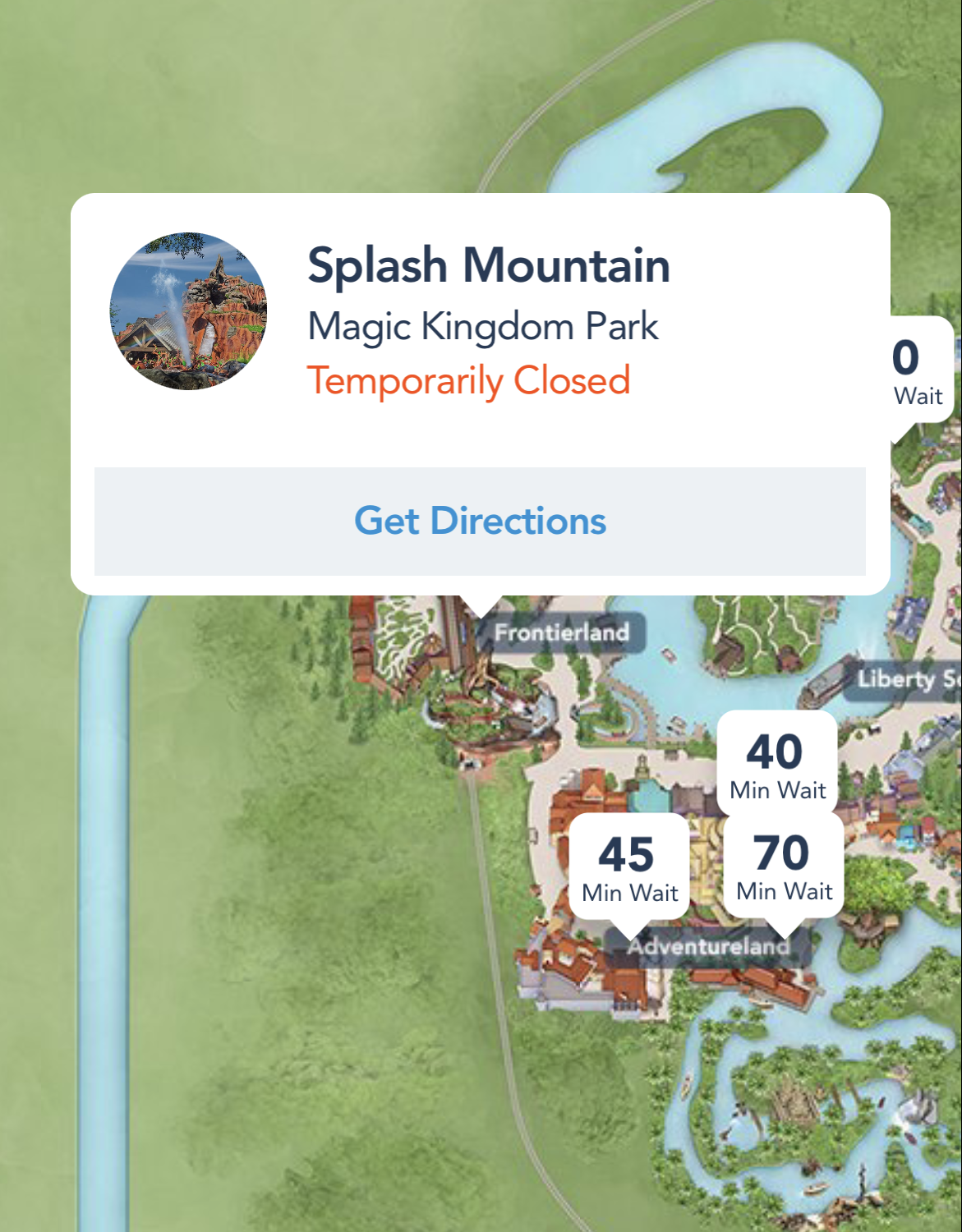The image is a screenshot from a mobile app displaying a map of a theme park, predominantly featuring green areas. A white rectangle overlay at the top indicates "Splash Mountain - Magic Kingdom Park - Temporarily Closed" along with an icon depicting Splash Mountain. An option to get directions is also visible. The background map shows various sections of the theme park, including Frontierland, Adventureland, and partially visible Liberty Square. A river flows from the bottom left corner, winding throughout the park. Notable wait times are indicated for several attractions within Adventureland, with signs showing 45-minute, 70-minute, and 40-minute waits. Another attraction to the north of Adventureland also has a wait time listed, but it is obscured by the white rectangle detailing Splash Mountain's closure.